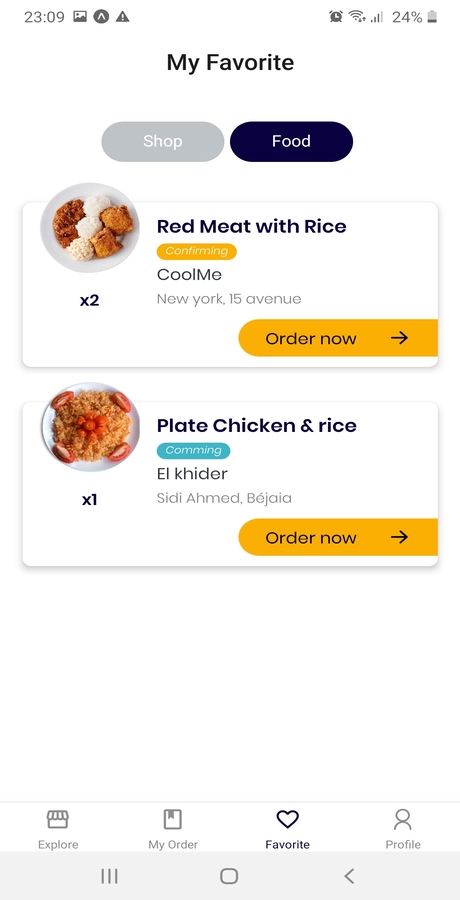This is a detailed screenshot from a mobile phone with a white background. In the upper left corner, various icons and information are displayed: the time is 23:09, followed by a photo icon, an A icon inside a circle, a triangle with an exclamation mark, an alarm clock, Wi-Fi signal, and mobile signal indicators. The battery level shows 24% with a corresponding icon.

Directly below, the screen presents a header that reads "My Favorite" in black font. Underneath, there are two buttons: a gray one labeled "Shop" and a navy blue one labeled "Food."

The main section features two entries. The first entry is titled "Red Meat with Rice," accompanied by a photo showing a plate of food that appears to include cauliflower and chicken nuggets. Below the photo, a yellow oval contains the word "Confirming." Further down, in black font, it states "Cool Me New York, 15th Avenue," accompanied by a yellow "Order Now" button with black text displaying "x2," indicating two orders of red meat with rice.

The second entry beneath this is labeled "Plate Chicken and Rice."